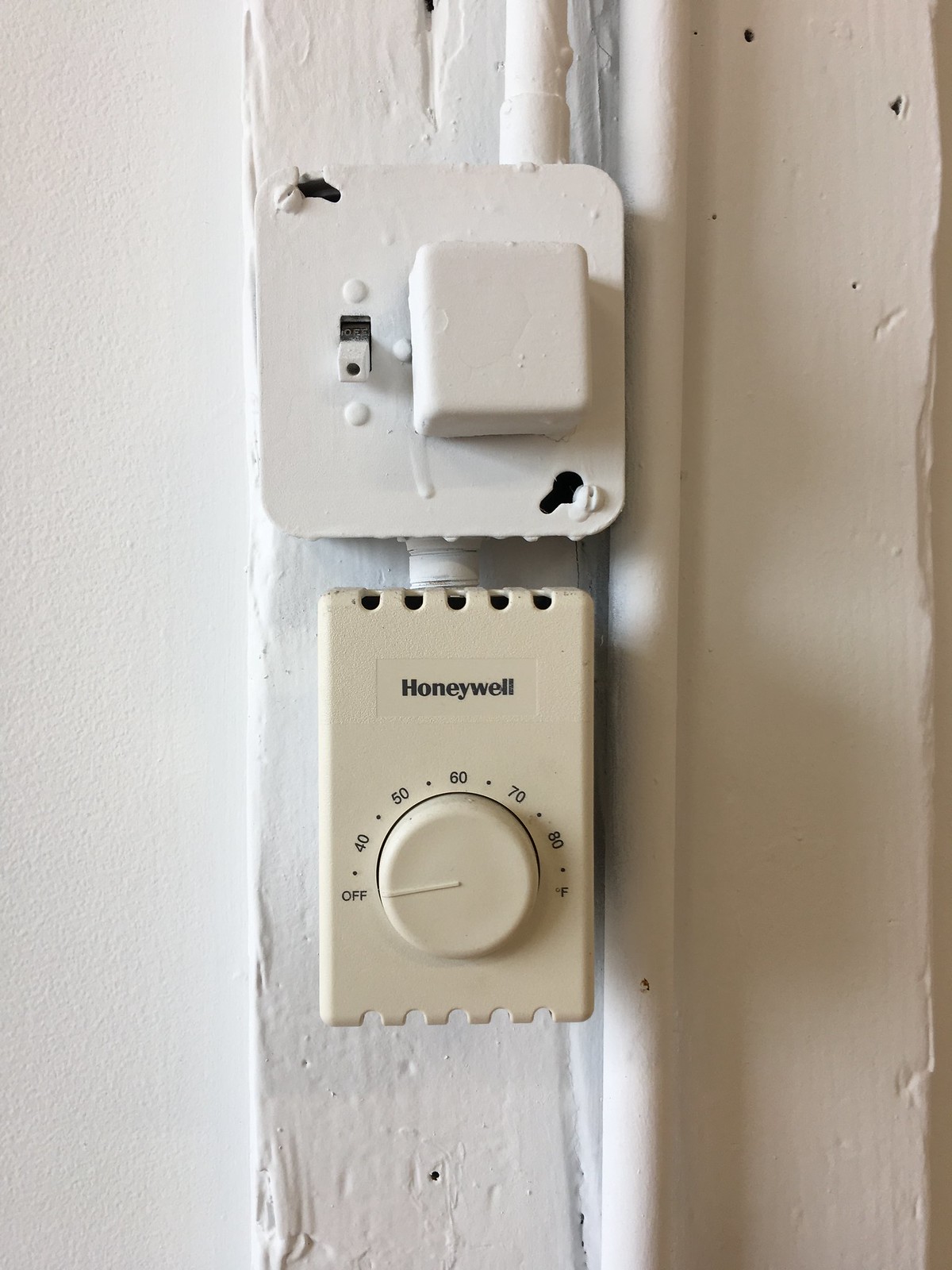On a white concrete wall, this image showcases a mechanical setup comprising several components. Dominating the center is a white two-by-four running horizontally, accompanied by small white pipes. One pipe runs vertically down the center of the image, while another descends from the top, ending about a quarter of the way down at a small light socket with a switch in the off position.

Mounted centrally on the wall is a square white electrical box, positioned just above an off-white Honeywell manual thermostat. The thermostat features a control knob and a temperature scale ranging from 'Off' to 40, 50, 60, 70, and up to 80 degrees Fahrenheit. The current setting of the thermostat's knob is in the 'Off' position, clearly indicating its status. This mechanical ensemble evokes a utilitarian aesthetic against the plain whitewashed wall.